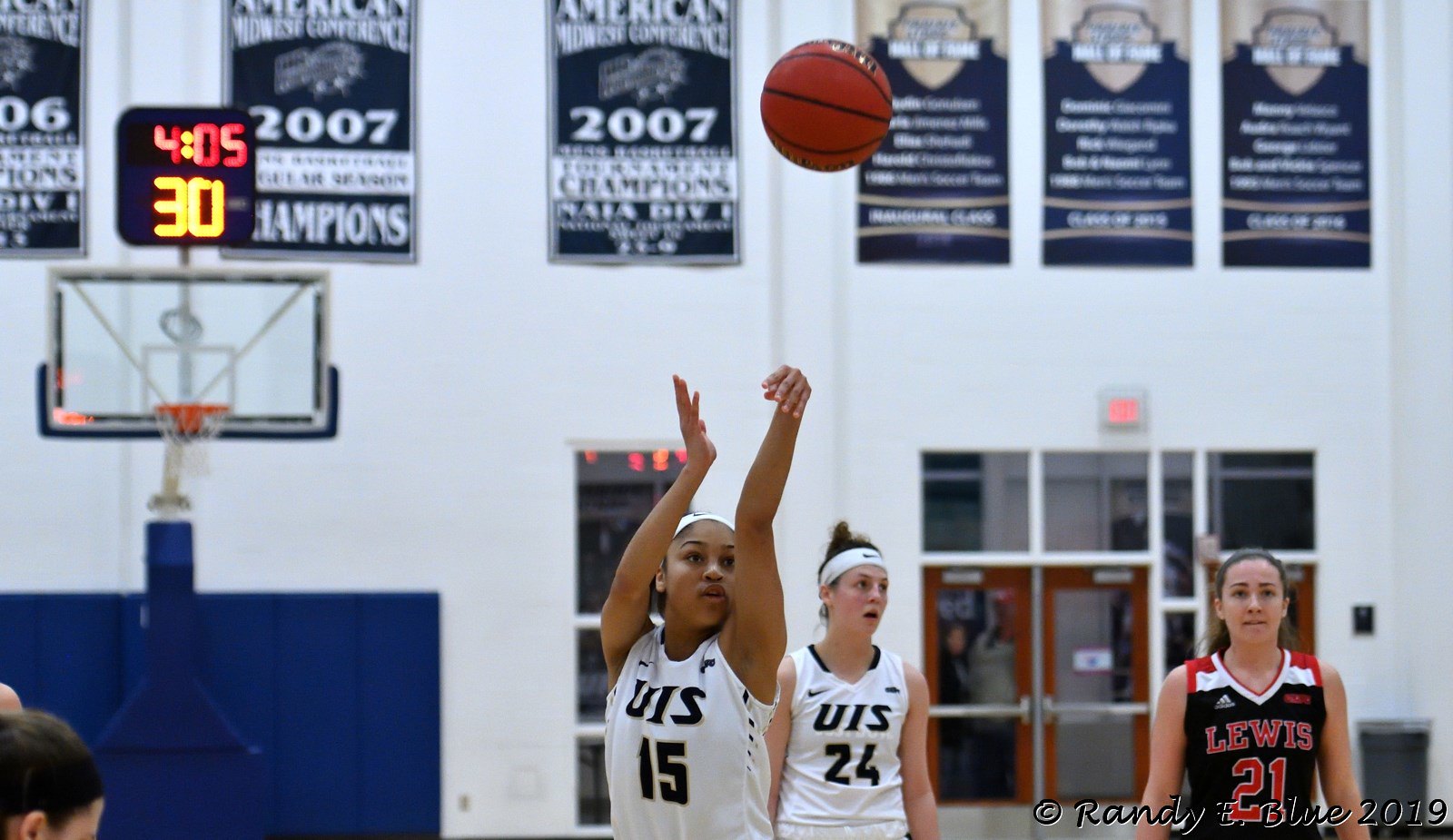The image captures a tense moment on an indoor basketball court, highlighting three players during a game. At the forefront is an African-American girl, intensely focused as she shoots a free throw. The orange basketball has just left her hands and is suspended mid-air. She is wearing a white jersey with "UIS" and the number 15, accompanied by a white Nike headband, her hair pulled back in a ponytail or bun. Behind her, a Caucasian teammate, also in a white jersey bearing the number 24 and a matching white Nike headband, can be seen. Both players are under the watchful eye of an opponent, who is clad in a black jersey with "Lewis" and the number 21. The background features white walls adorned with banners and posters displaying various years, including 2007 and an incomplete 06, indicating past successes or events. Additionally, a red-lit scoreboard above the net indicates 4:05 on the timer and a score of 30. The corner of the image bears a label, "randye.blue2019," perhaps marking the photo's origin or the photographer.